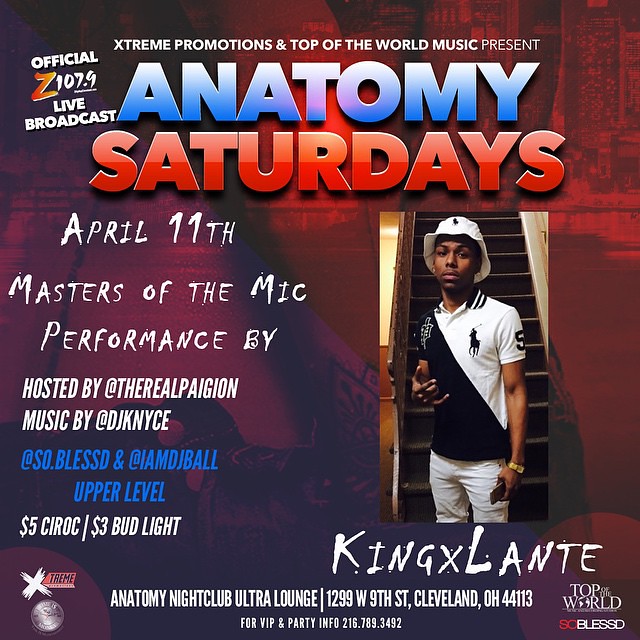This is a detailed advertisement flyer for a music event titled "Anatomy Saturdays," featuring a vibrant red background with black highlights. At the top, it announces, "Extreme Promotions and Top-of-the-World Music Presents Anatomy Saturdays," with "Anatomy" written in blue and "Saturdays" in a glossy red font. The flyer highlights that the official Z107.9 live broadcast will take place on April 11th. 

The central image showcases an African-American male standing in front of a staircase, donning white pants, a black and white polo shirt with a polo player emblem, and a matching white hat. He accessorizes with a gold watch on his right wrist and appears to be holding a cell phone in his raised right hand. 

The event features performances by King Xlante (stylized as K-I-N-G-X-L-A-N-T-E) and is hosted by @TheRealPagan, with music by @DJNice, @SoBlessed, and @IAMJBall. Additionally, the flyer notes promo deals including $5 Ciroc and $3 Bud Light on the upper level. 

The venue for the event is Anatomy Nightclub Ultra Lounge, located at 1299 West 9th Street, Cleveland, Ohio 44113. For VIP and party information, attendees are encouraged to call 216-789-3492. Social media links and further event details populate the left side of the flyer.